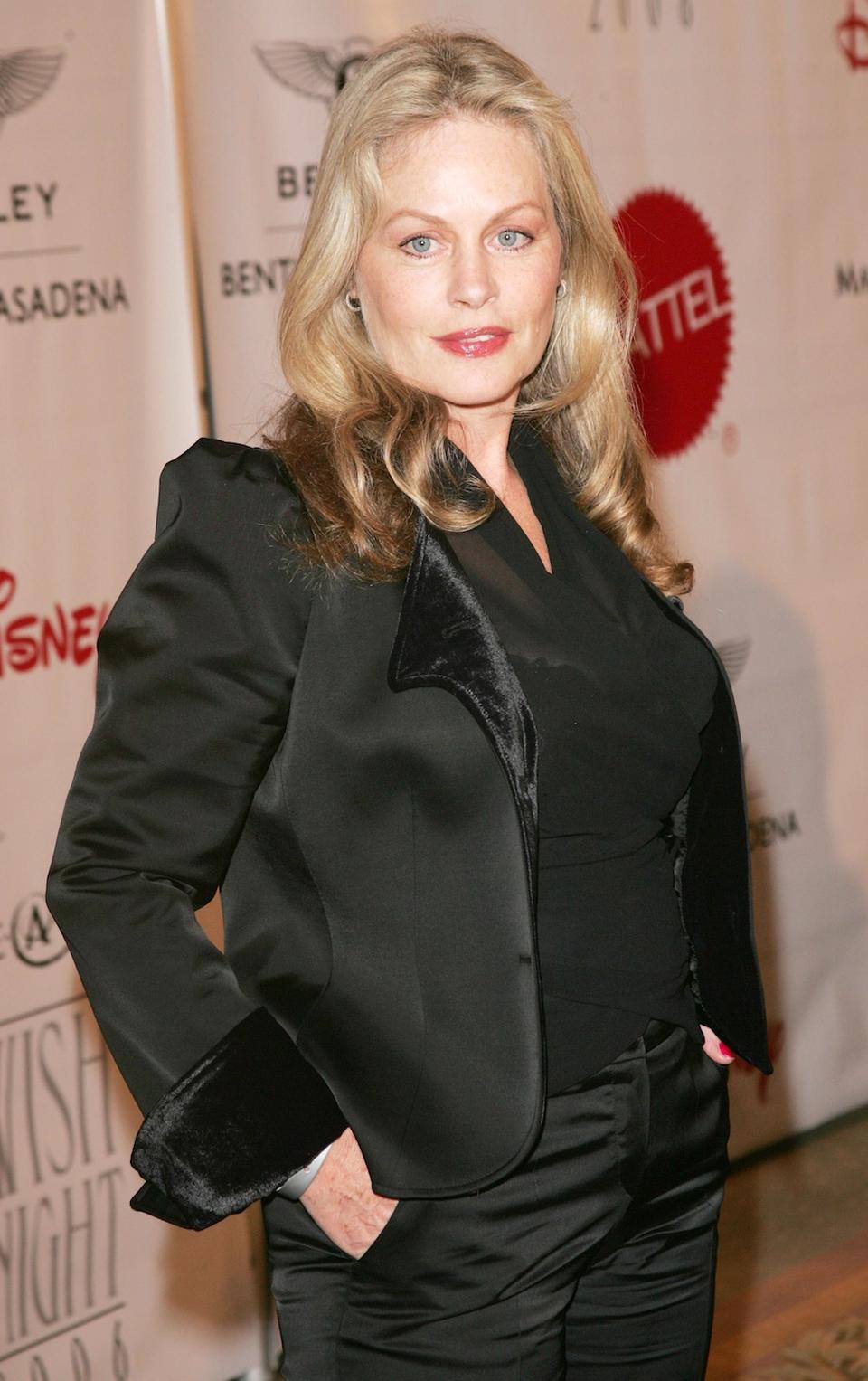This photograph captures a blonde-haired, white female who appears to be a celebrity posing on a red carpet. She is dressed in an all-black ensemble that includes a black blouse underneath a velvet-blazer with satin-like cuffs and lapels, complemented by black satin pants. Her long, blonde hair cascades past her shoulders, and she has light blue eyes. Small hoop earrings can be seen adorning her ears, and she has her hands tucked into her pants pockets as she gazes slightly to the left. The background is a white wall adorned with several company logos, including a partial view of Disney in red, the Mattel logo in a red circle, and part of a Bentley Pasadena logo. The image itself is narrow and closely cropped, focusing primarily on the woman, with minimal background details.